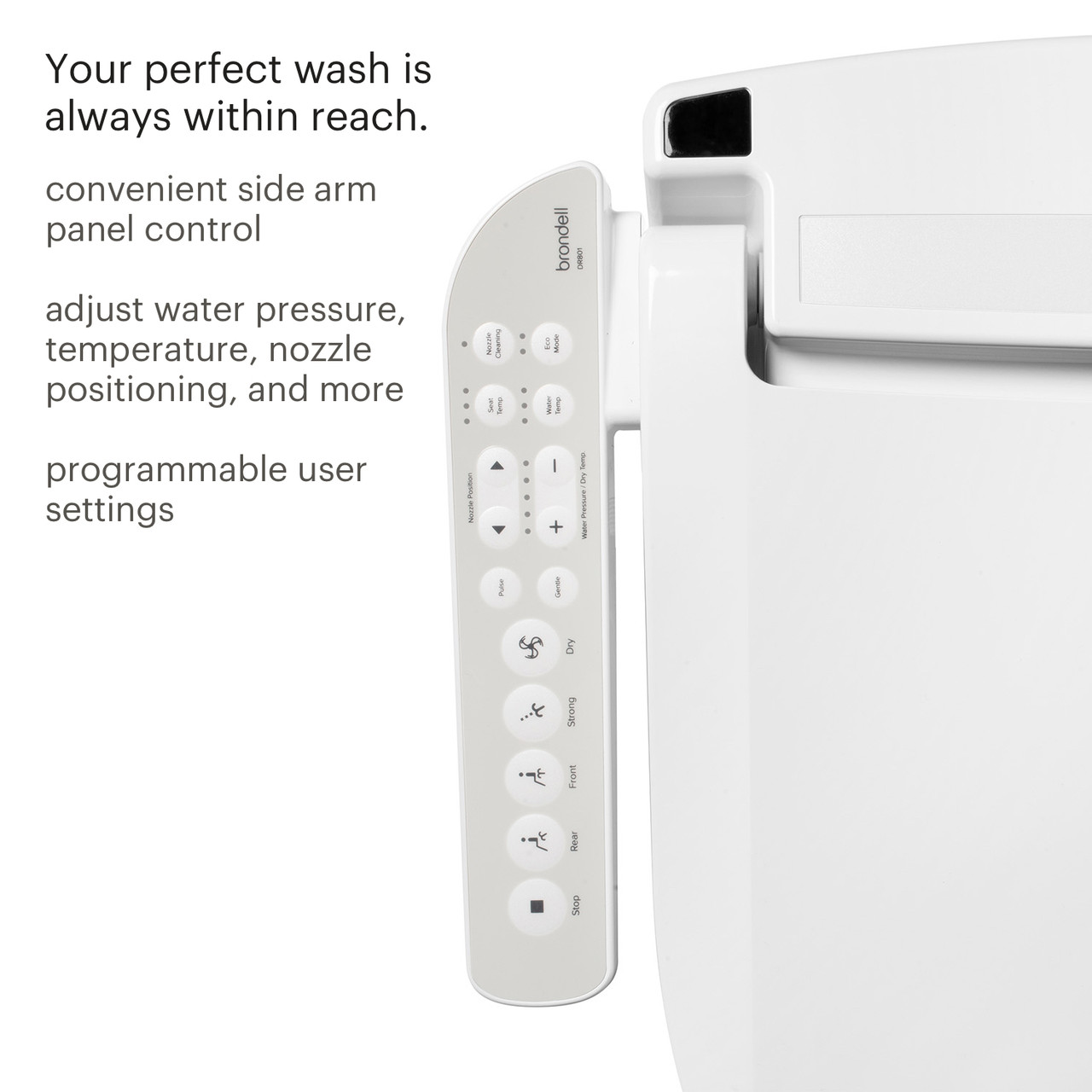The image is a vertical advertisement for a Brondell bidet toilet seat, specifically highlighting the left section of the seat. The photograph showcases the seat's side control panel coming in from the right, complete with a distinctive hinge and a small sensor. The white bidet features soft-touch push-button controls that are slightly raised from the surface. These buttons display various icons, such as individuals in different seating positions, jet streams, and a fan, indicating it has a drying function. The controls also include up and down arrows and plus and minus symbols, likely for adjusting heat or water pressure, although the specific details are not legible.

The right side of the image is a stark white photograph set against a brighter white background, drawing attention to the sleek design of the bidet. The left side features black text that reads, "Your perfect wash is always within reach. Convenient sidearm panel control adjusts water pressure, temperature, nozzle positioning, and more. Programmable user settings." This description suggests a user-friendly device with customizable options for an optimal experience.